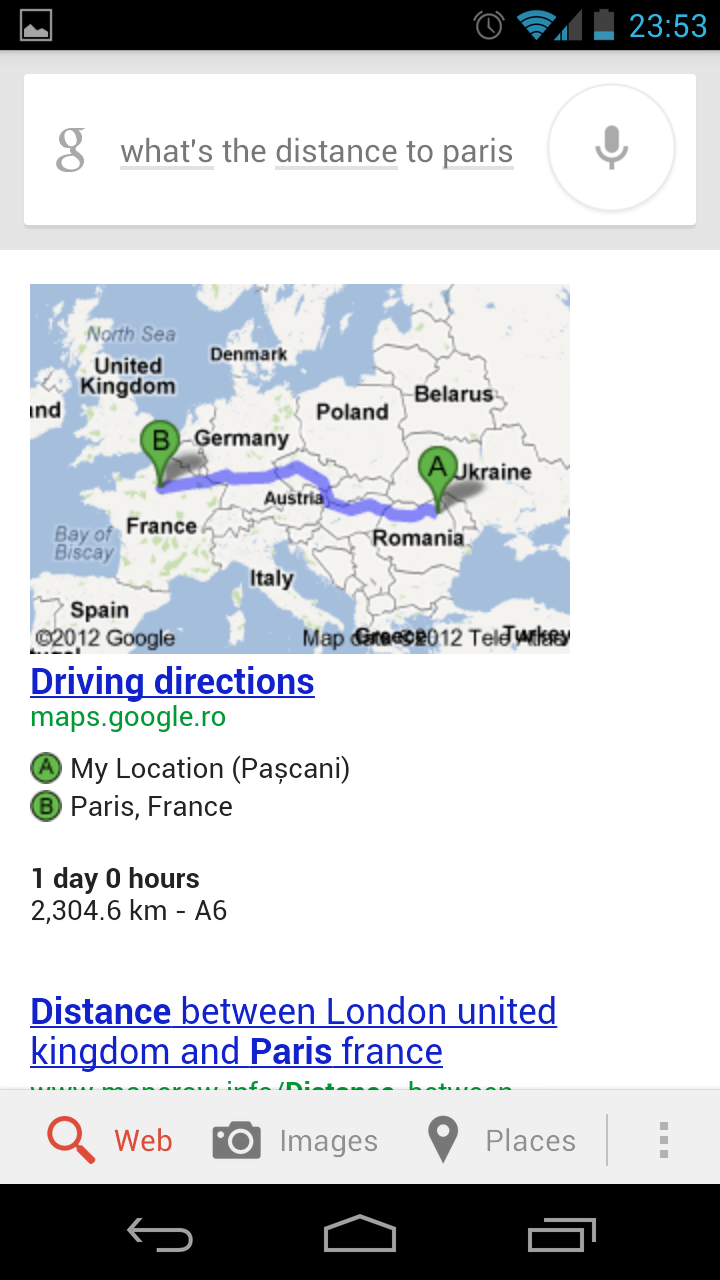The image is a screenshot of a Google search results page, specifically highlighting a query for the distance to Paris. In the search bar at the top, the text reads, "What's the distance to Paris," flanked by the Google "G" logo on the left and a microphone button on the right. 

Below the search bar is an interactive map showing a route from Point A, located in Pascani, Romania, to Point B in Paris, France. A blue line indicates the driving path between these two points. 

Under the map, the text reads "Driving directions" with the link to "maps.google.ro." The starting location (Point A) is listed as "My location, Pascani" and the destination (Point B) as "Paris, France." The driving distance is noted as "1 day, 0 hours" and covers "2,304.6 kilometers." The A6 is mentioned, likely referring to the highway used in the directions.

Below this information, additional search results include the text "Distance between London, United Kingdom and Paris, France." 

At the bottom of the screen, there are various search filter buttons: a magnifying glass labeled "Web," a camera labeled "Images," a pin icon labeled "Places," and a menu icon with three vertical dots. The standard phone navigation buttons (back arrow, home button, and recent apps button) are also visible, indicating this is a mobile device screenshot. The numerical figure "2353" appears at the very end, though its relevance is unclear from the context.